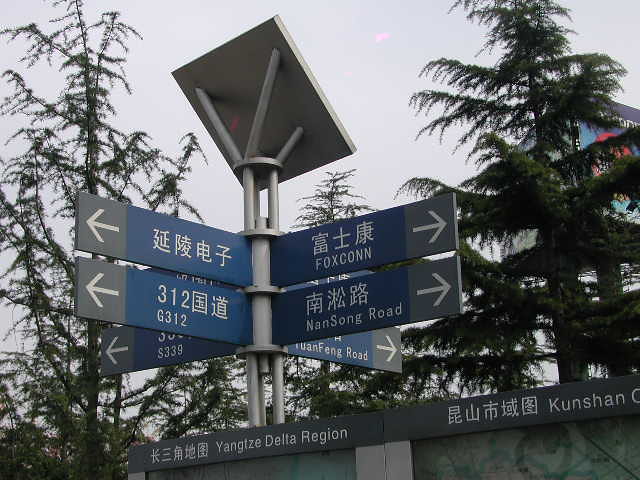This photograph captures a detailed scene at a multi-directional intersection in China. Dominating the image are several blue street signs featuring Chinese characters and directional arrows pointing in various directions. The prominent signs include one indicating "Foxconn" and another naming "Nansong Road," both directing to the right. Another sign directs to the left with the designation "G312," accompanied by additional Chinese characters. Underneath, a further sign at the bottom reveals the text "Yangtze Delta Region," while another section includes "Kunshan" before being cut off. Adding to the complexity of the scene, the signage structure appears to incorporate a solar panel and possibly connects to a nearby bench displaying advertisements. In the background, green trees and a grey sky provide a contextual outdoor setting for this bustling intersection.